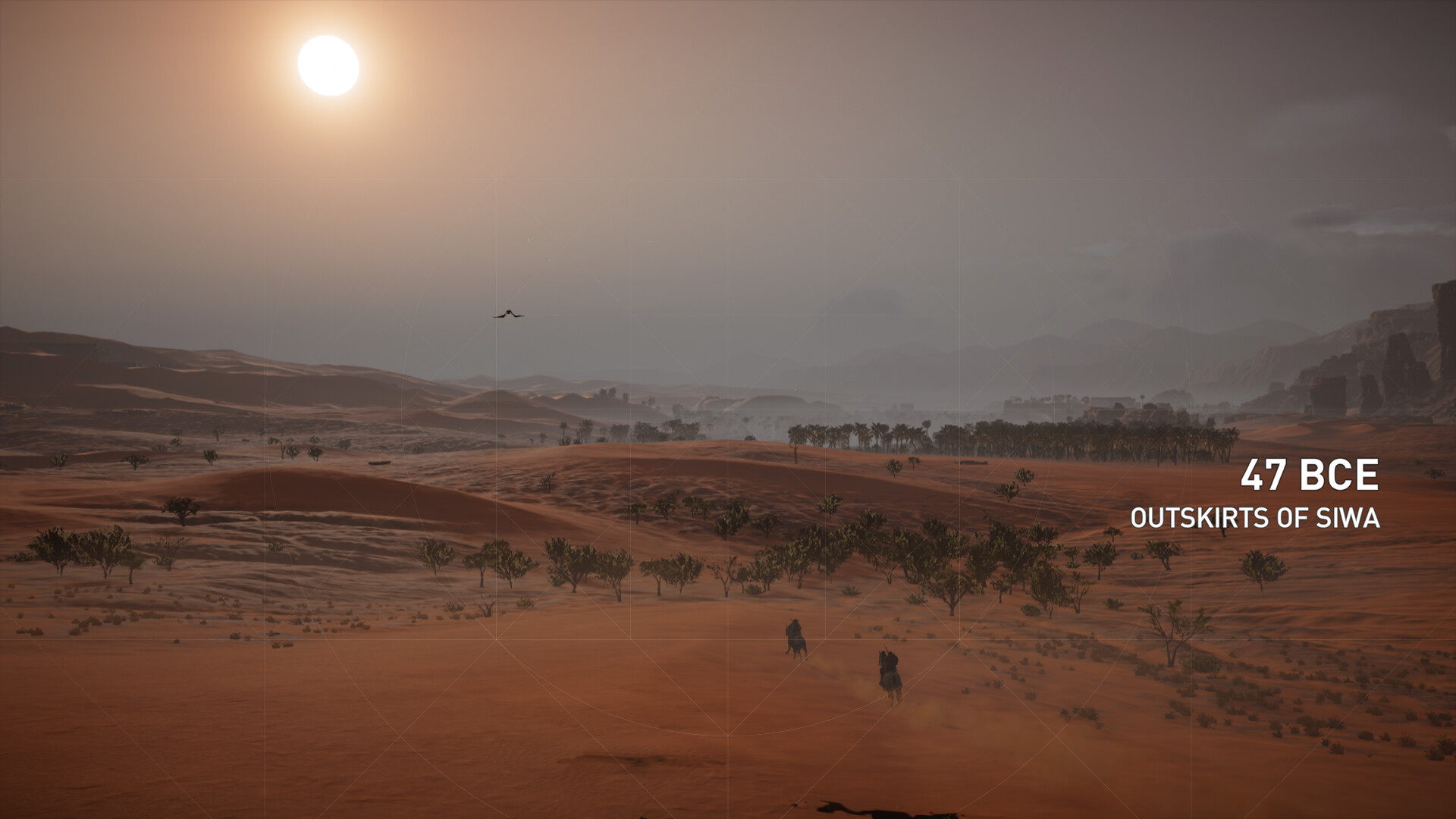This daytime photograph captures the arid landscape of the outskirts of Siwa, dated to 47 BCE. The scene is dominated by an expansive desert, with fine, red sand stretching endlessly across the terrain. Sparse tufts of hardy desert trees break the monotony, alongside gentle undulations that hint at distant hills. In the lower part of the image, two figures on horseback are visible, their backs turned as they journey towards the center, becoming small silhouettes against the vast sandscape. High above, a solitary bird soars across the sky near the upper left corner of the frame. The warm sun, partially veiled by a diffuse haze, lends a soft, golden glow to the scene, enhancing the austere beauty of the desert environment.